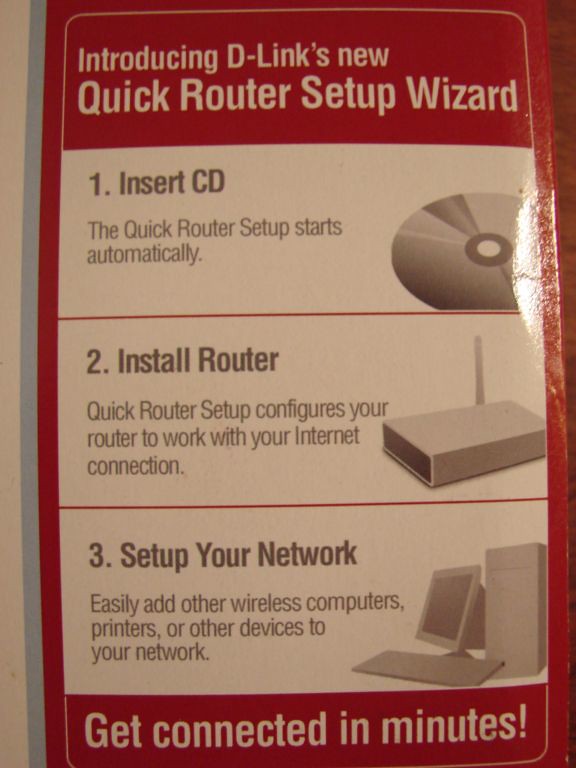The image showcases a rectangular instructional guide from D-Link, predominantly featuring a glossy red and white color scheme, designed to facilitate a quick router setup. At the top, bold white text introduces "D-Link's new Quick Router Setup Wizard." Below this, three sequential instructions are displayed in white rectangular boxes accompanied by grayscale clipart. The first box instructs to "1. Insert CD," with an image of a CD, noting that the Quick Router Setup will start automatically. The second box directs to "2. Install Router," illustrated by a router image, explaining that the setup configures the router to work with your internet connection. The third box instructs to "3. Set up your network," depicted with a computer monitor clipart, indicating that you can easily add other wireless computers, printers, or devices to your network. At the bottom, a red banner with white text reassures users: "Get connected in minutes." The guide's clean design and clear instructions make it simple and attractive to read, ensuring an easy-to-follow router setup process.